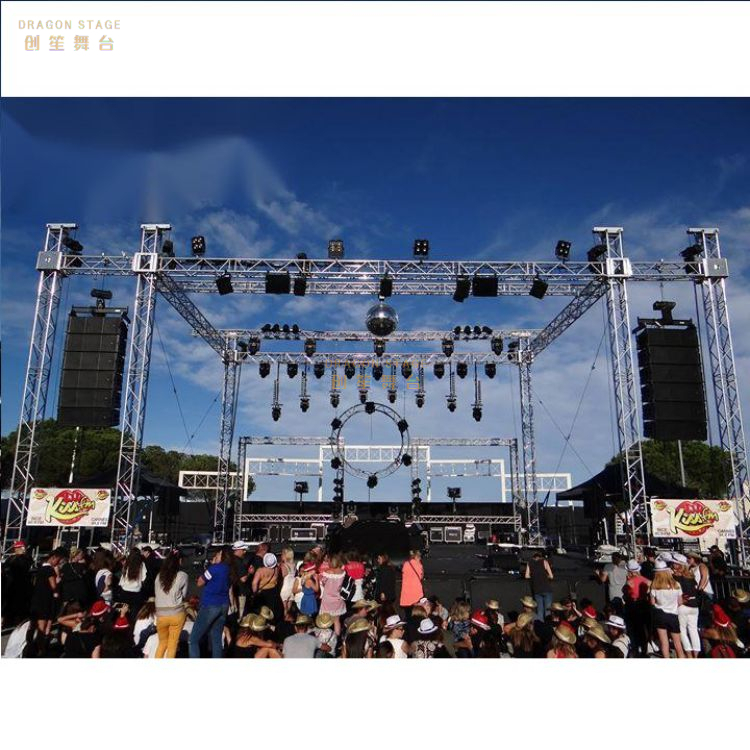The image captures a vibrant and bustling outdoor concert setting on a sunny day with a clear blue sky and scattered white clouds. At the center of the image is a large, metal stage adorned with tall poles and black lights. The stage, which has a black platform, features prominent signage on both sides, displaying the KISS FM logo with a pair of lips in the background on a pink backdrop. Additionally, there is beige-colored text reading "DRAGON STAGE" at the top left, accompanied by traditional Chinese characters. The crowd in the foreground, consisting of both seated and standing spectators, appears eagerly poised to enjoy the concert. The natural backdrop includes green trees and leaves visible on both the left and right sides, enhancing the summery and festive atmosphere. Yellow cursive text further decorates the setup, contributing to the cheerful and engaging ambiance of the event.